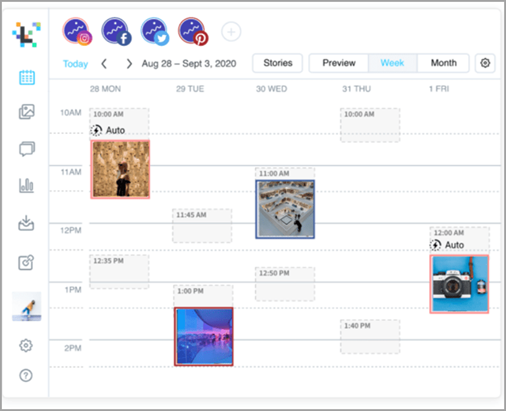Screenshot of a digital calendar interface covering the week of August 28 through September 3, 2020. The top of the calendar displays navigation options such as "Today," "Stories," "Preview," and different viewing modes, with "Week" currently selected. Days of the week are listed in columns from "Monday 28" to "Friday 1" along the top. Time slots are prominently shown, ranging from 10 a.m. to 3 p.m., followed by scattered labelings like 10 p.m., 11:45 a.m., 12:35 p.m., 12:50 p.m., and ending at 1:40 p.m. The screenshot is purely focused on the calendar interface without any illustrations, animals, plants, buildings, banners, signs, vehicles, or bicycles depicted.